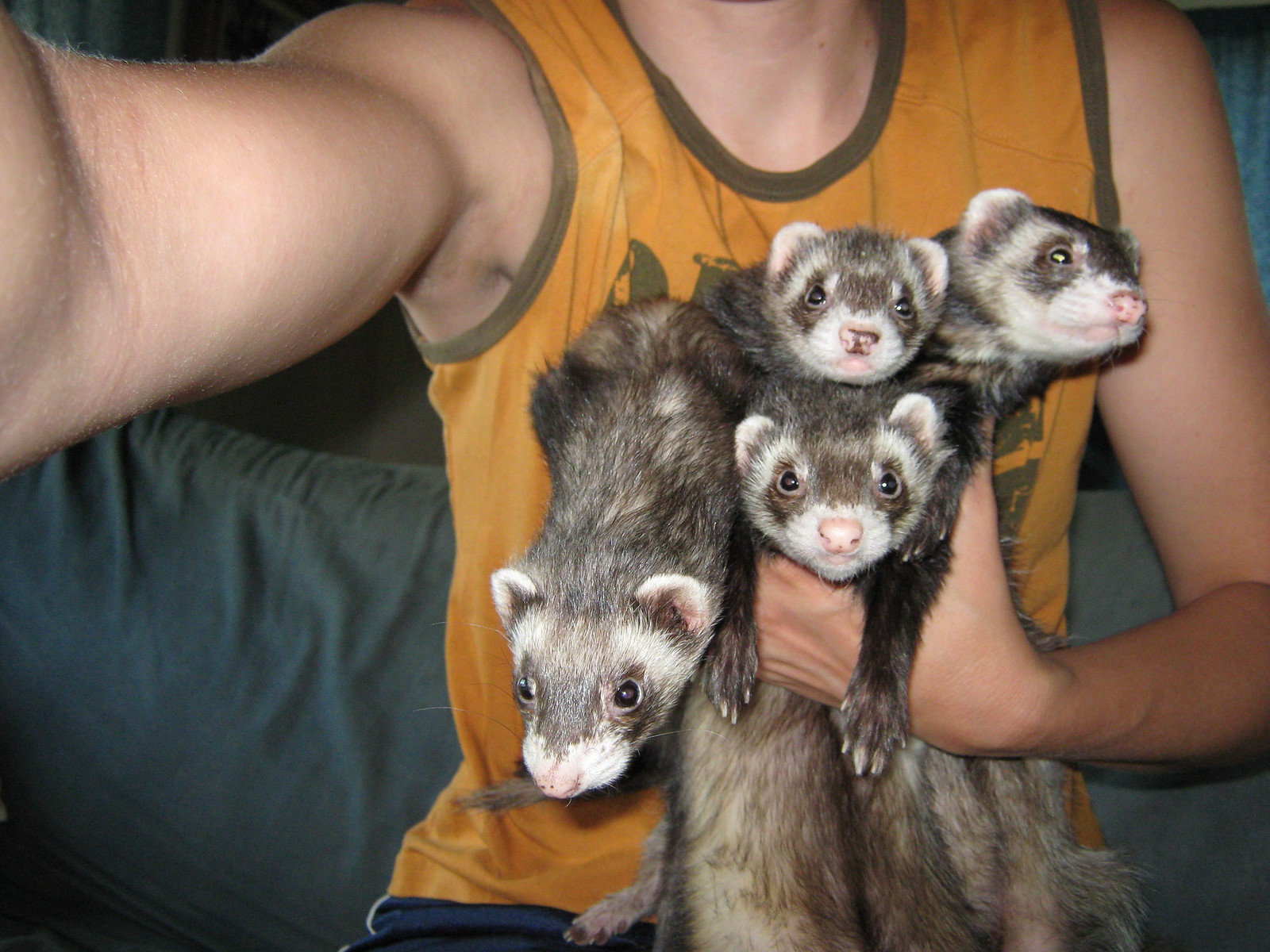This color photograph, taken in landscape orientation, appears to be a selfie captured with a flash in an interior setting. The left side of the image shows the individual's arm extended outward, presumably holding the camera. The person is wearing an orange tank top with greenish-brown trim around the armholes and neck. The individual’s head is cut off from the neck upwards, making it impossible to see their face. 

Their right arm is bent at a 90-degree angle, holding four ferrets against their chest. The ferrets all have dark brown fur with lighter streaks and lighter colored stomachs. They each exhibit white patches around their nose, with the majority having pink noses and one displaying additional brown markings. The ferrets also have white perimeters around their ears. The animals are draped over the person's hand, appearing relaxed and slouched, almost like they're slumping over his hand.